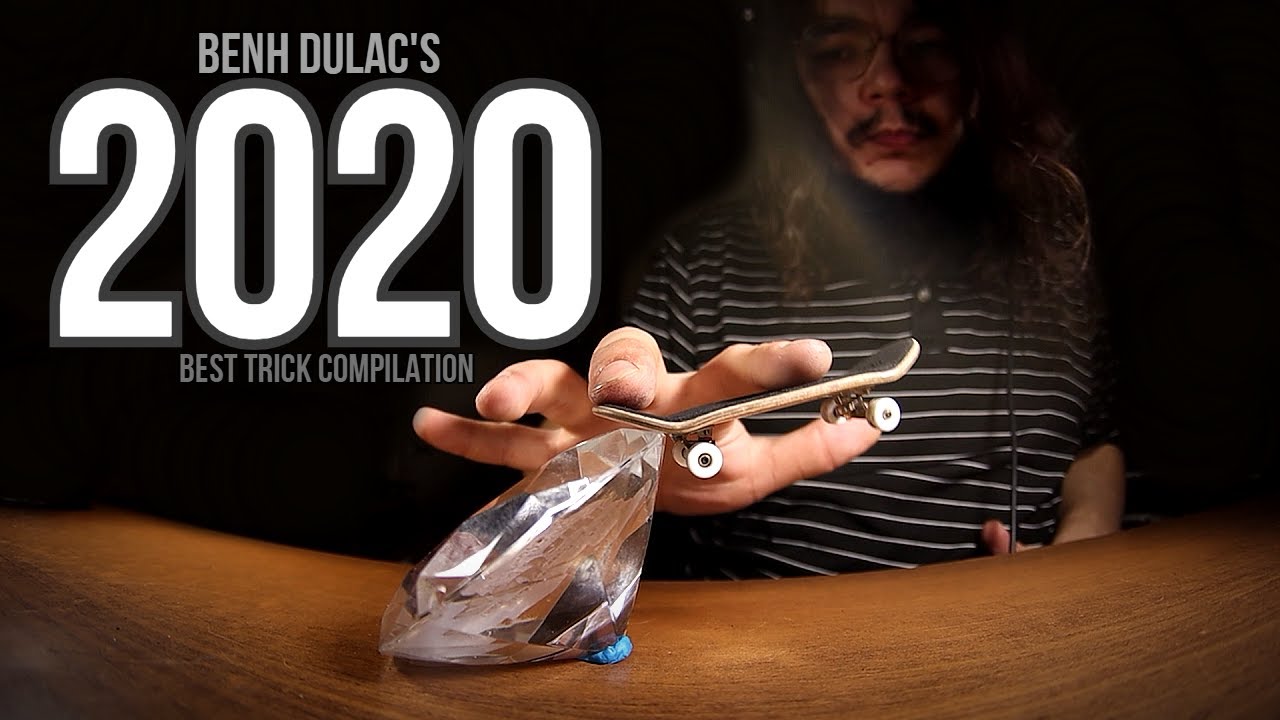A detailed caption for the image could be:

"In this striking image, a man with long dark brown hair, a distinct mustache, and glasses is shown mainly in darkness. He dons a black shirt adorned with white horizontal stripes and is intensely focused on performing a trick with a miniature skateboard, known as a tech deck. This tiny skateboard is positioned very close to the camera, executing a trick on a large, intricately carved plastic diamond with a blue, squishy base. The bottom section of the image displays a wooden table, seemingly warped, possibly due to a fisheye lens effect, while the backdrop remains stark black. In the upper left section of the image, bold text reading '2020' is prominently bordered in gray, occupying about a fourth of the image. Above '2020,' in smaller font, it reads 'Ben Dulack' (spelled B-E-N-H-D-U-L-A-C), and underneath, 'Best Trick Compilation' is inscribed in very small font. The overall composition hints that this could be a thumbnail for Ben Dulack's 2020 Best Trick Compilation video."